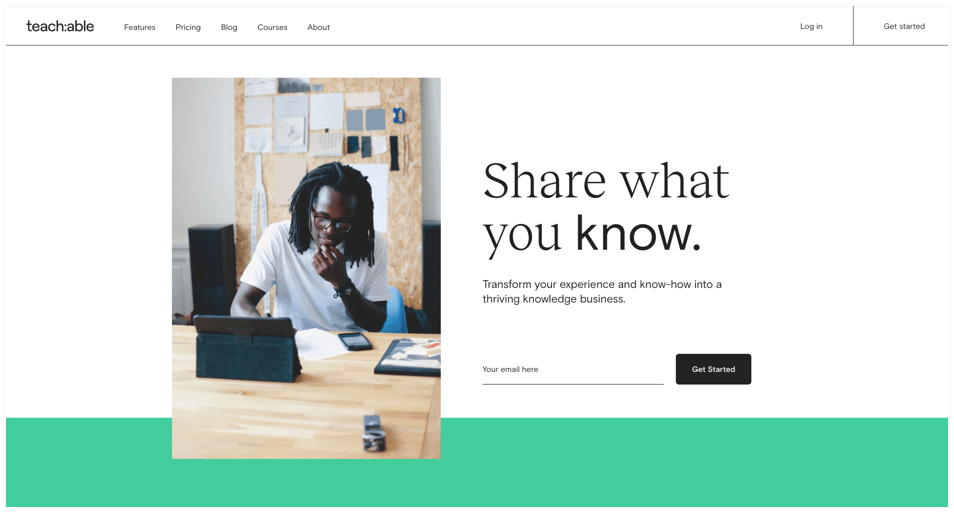A minimalistic website, "Teachable," showcases a clean design with a navigation bar at the top featuring sections such as Features, Pricing, Blog, Courses, About, and options for Login or Get Started. Dominating the center of the page is a stock photo of a young Black man with dreadlocks, seated at a desk that could be in either a formal office or a home office. He wears glasses and a wristwatch, with his hand thoughtfully placed against his chin. In front of him on a light wooden table are a phone, a piece of paper, and a tablet propped up on a stand. Beside him, the text reads "Share what you know," followed by "Transform your experience and know-how into a thriving knowledge business." Below this is a field to enter an email address and a black "Get Started" button. The rest of the page is predominantly white, accentuated by a green horizontal band at the bottom for a touch of color.